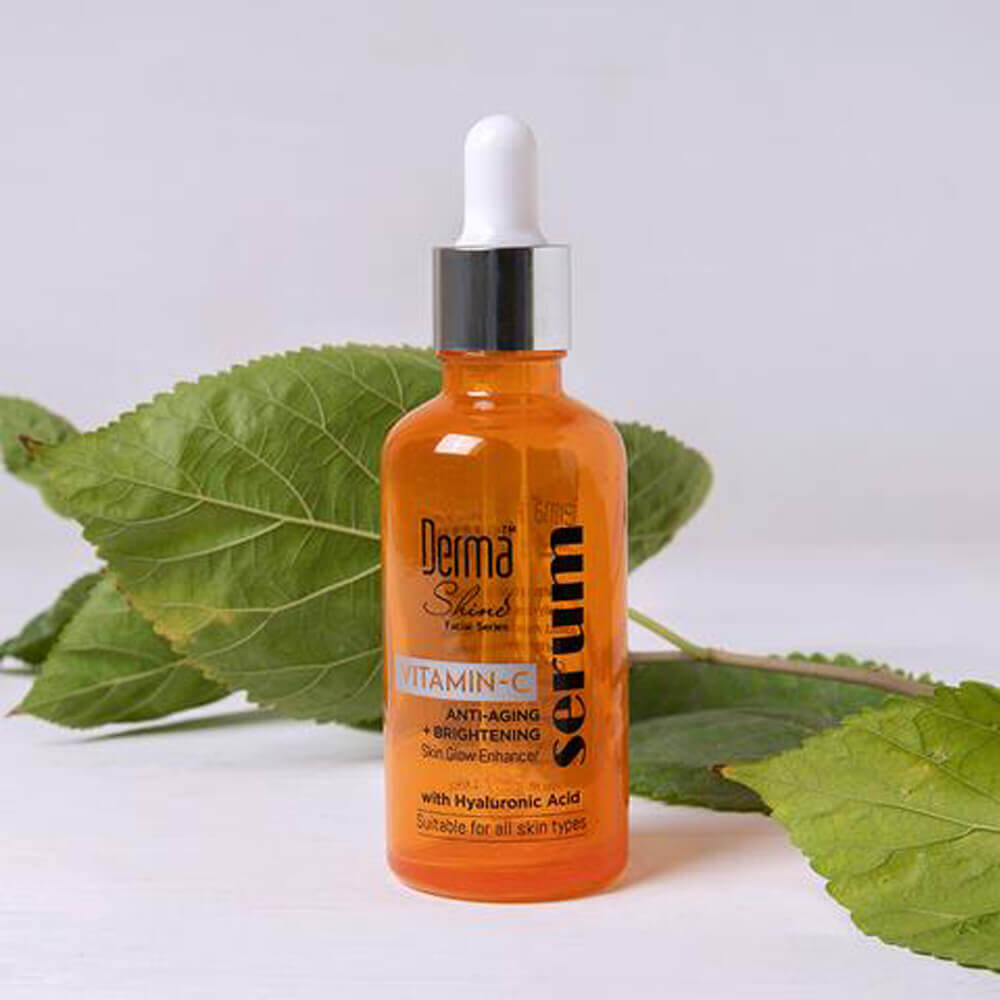The image features a small, plastic vial of serum with an orange liquid inside, prominently displayed in the center. The vial is labeled with "Dermashine" in black letters, followed by "Vitamin C" in orange letters on a gray background. Below this, in black text, it reads "anti-aging and brightening", "skin glow enhancer", and "with hyaluronic acid". To the right, the word "SERUM" is written vertically in bold black letters. The vial has a silver cap with a built-in dropper, ending in a rounded white tip. 

The backdrop is a solid medium gray square, creating a neutral yet striking background. Adding depth to the composition, large, defined green leaves occupy the middle and lower right corner, their veins and textures clearly visible. Some of the leaves display brown spots and visible stems, enhancing the natural aesthetic of the scene.